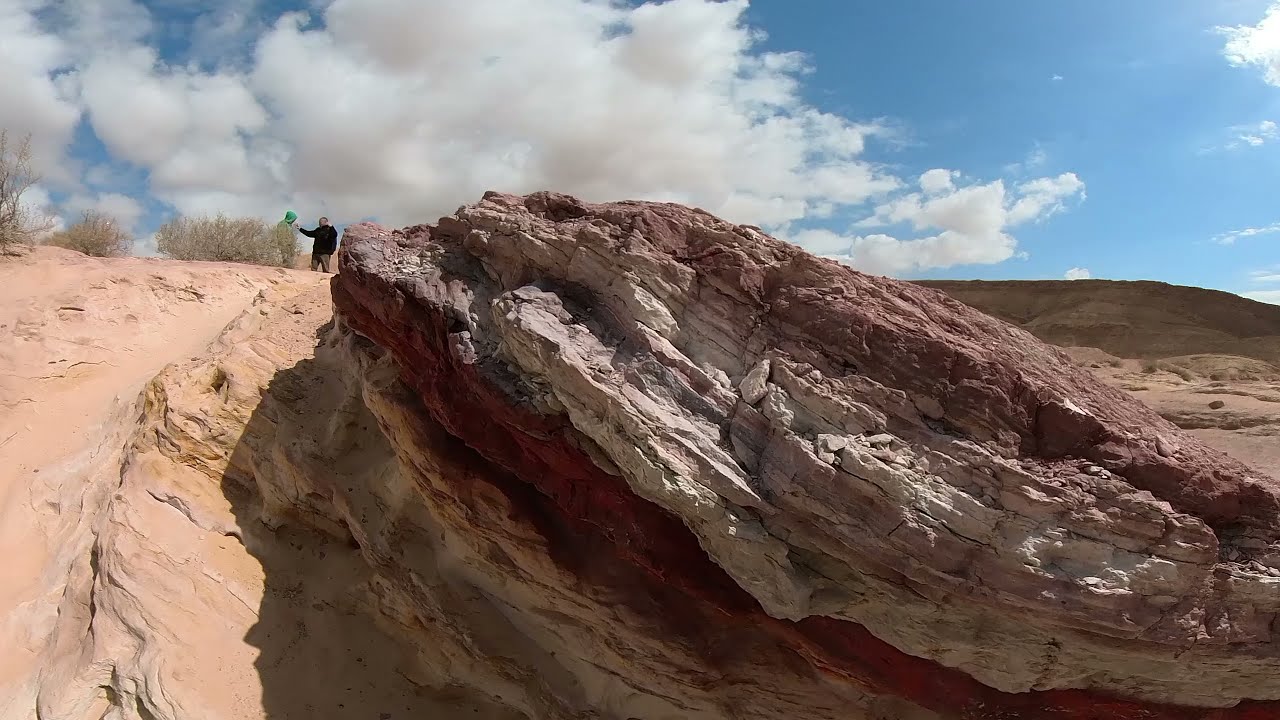The image captures a broad view of a canyon-like landscape featuring two men. The terrain is divided into two distinct rock formations. The left side displays a smoother, light brown rock surface that transitions to gray and condenses in certain areas. In contrast, the right side boasts a jagged multicolored rock face with layers ranging from light brown at the top, white in the middle, reddish-brown below that, and orange at the base; this structure casts a shadow on the smoother rocks to the left. Atop these formations stands one man wearing green pants and a black sweatshirt, while another man in a bright green hoodie can be seen behind a small green bush. Above, a vibrant blue sky with a large white cloud dominates the top of the image, highlighting the outdoor daytime setting. The contrasting colors of the rocks—from pink and rust-red to various shades of brown, beige, and gray—along with the vivid sky, add depth and rich detail to this canyon scene.